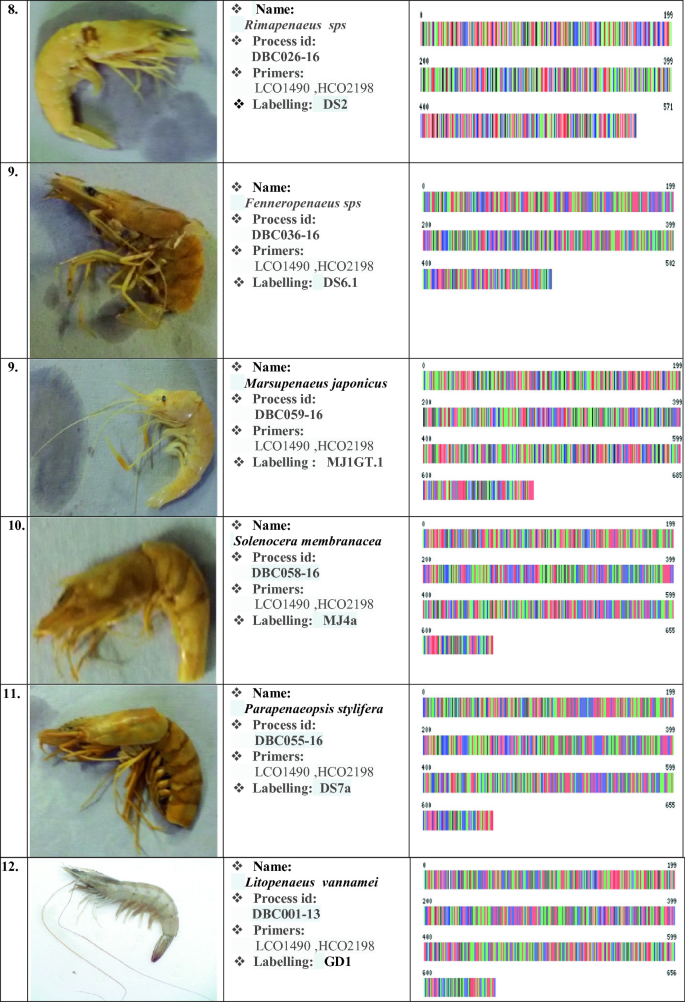The image is a detailed, multi-part chart displaying six different types of shrimp or similar organisms, numbered sequentially from 8 to 12 along a thin vertical strip on the left side. Adjacent to each number is a square panel containing identifiable images of the organisms: the top five pictures appear as colored photographs on a gray background, while the sixth image, at number 12, stands out with a smaller, whitish appearance on a white background, resembling a larva or a drawing. To the right of each image, a white box provides detailed information, including the name of the species, process ID, primers, and labeling. The rightmost section of the chart is occupied by a large rectangular box filled with rows of small, colorful vertical lines, reminiscent of a stylized barcode using red, green, purple, and blue hues. Each organism's data is followed by three to four rows of these brightly colored lines, providing a complex and visually engaging representation.